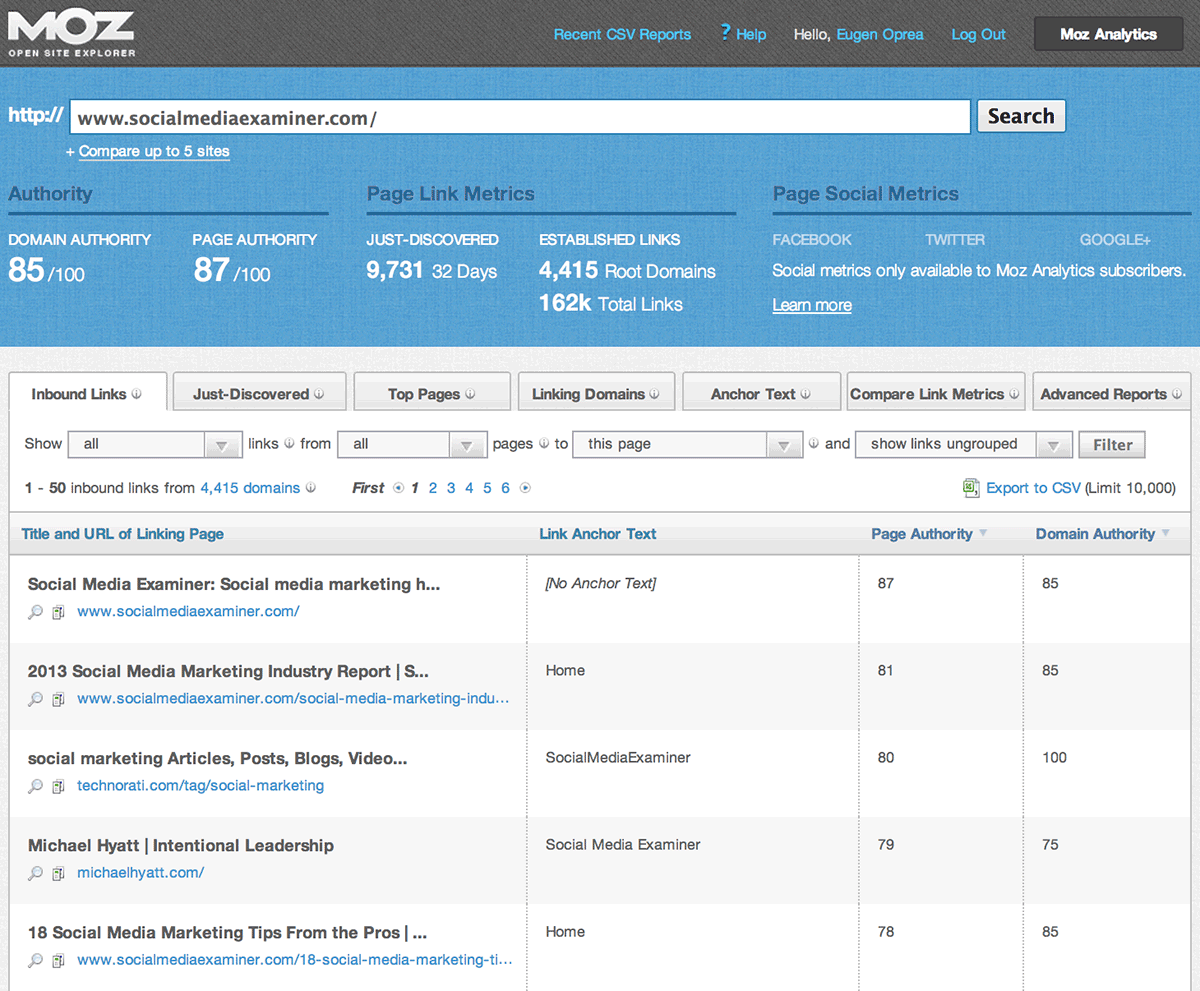The image features a user interface displaying a search engine results page. In the top left corner, the white letters "M-O-Z" stand out against a black background. On the far right side of the top section, there are additional words in blue and white text. 

Below this, a white search bar is set against a blue background, with black and white text underneath it. The lower portion of the image has a gray background, featuring black text. 

At the bottom of the page, there's a section that appears to be a table or graph, likely representing search results. This area includes blue navigation links for multiple pages, labeled from "page one" to "page eight." Each search result entry includes a blue URL beneath a black title. On the far right side, the text reads "Flip Rewards Sovon Kilvichur."